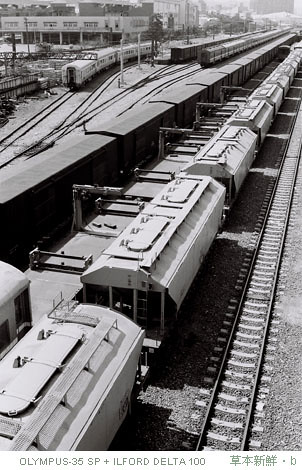The photo in question is a detailed black and white image of a train yard, taken from an elevated viewpoint. Across the bottom of the image, there are grey text inscriptions reading "Olympus 35 SP" and "Ilford Delta 100," accompanied by Japanese characters and a dot followed by a "B". 

The yard comprises six railway tracks, captured with notable clarity. On the rightmost track, a segment of railway is devoid of any trains. Adjacent to this, on the second track from the right, resides a cargo train carrying white, rounded containers which feature air openings on top, reminiscent of exhaust pipes.

Further to the left, what initially appears as a platform laden with metallic pieces is actually the roof of another parallel train. This train consists of a flatbed car, with a larger car extending from the bottom left. To the far left of this, an even darker train sits on the tracks, characterized by standard box cars with black sides and white roofs.

In the background, the rail yard continues, showing additional railway lines. Two more trains are visible on the left, and a white train curves off to the left side, providing a sense of depth to the scene. The yard is bathed in sunlight, casting distinct shadows of the trains onto the ground. Distantly, a large building looms over the yard, indicating a possibly significant structure, likely related to operations or administration. Sparse human figures are scattered, emphasizing the industrial bustle of the scene.